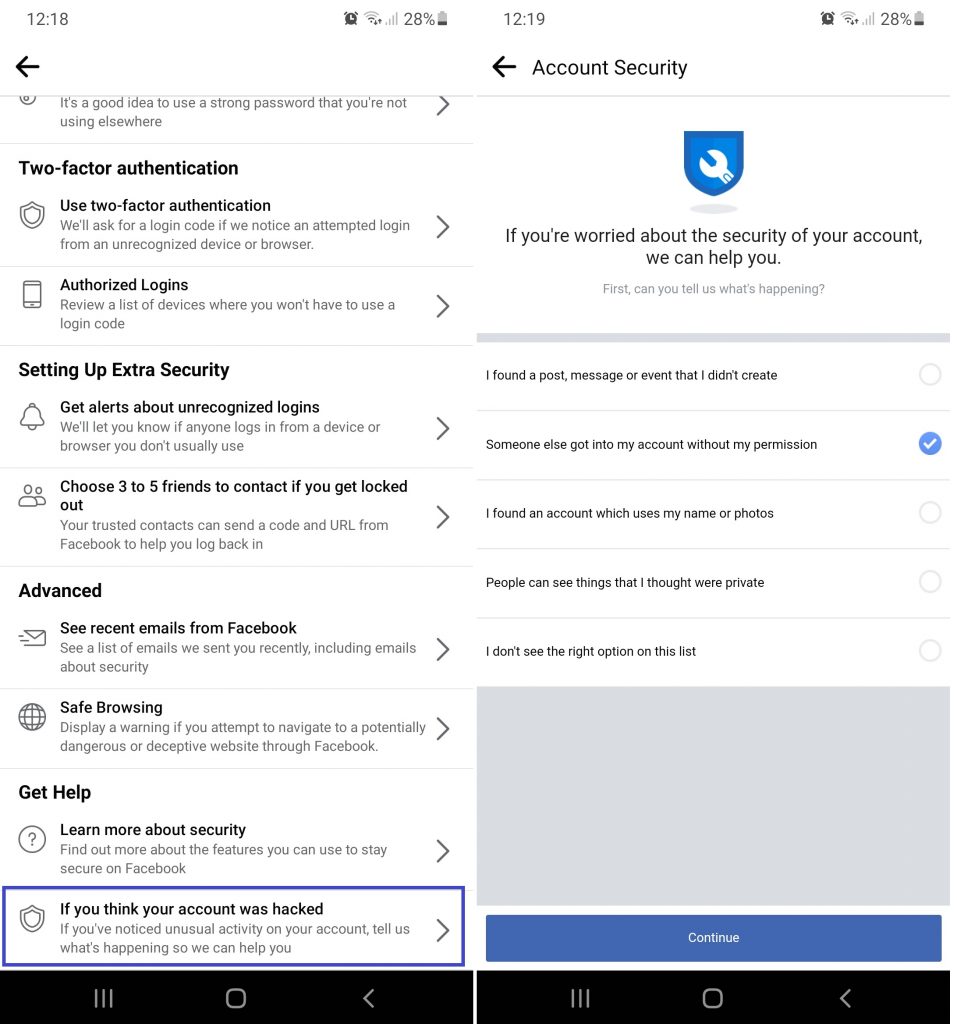**Descriptive Caption:**

In the upper left corner (12-15 o'clock position), there is a prompt suggesting the use of 2% energy with a 28% electro setting. It highlights the importance of enabling two-factor authentication for enhanced security. This feature will prompt you for a login code if it detects an attempt to log in from an unrecognized browser. There is a comprehensive list of devices such as smartphones and Wii consoles where you don't want to bypass this security measure. By setting up extra security, you receive alerts about any unrecognized logins, ensuring you're informed if someone tries to access your account from an unfamiliar device or browser. 

You can choose 3-5 trusted friends to help you regain access to your account should you get locked out; these friends can send you a security code from Facebook to assist you in logging back in. The image also shows recent emails from Facebook, including those related to account security, demonstrating a secure browsing experience and the importance of monitoring potentially dangerous sites through Facebook.

Further security features and educational resources are available, guiding you to learn more about how to protect your account. In case your account is compromised, there is an option to report unusual activity, such as posts, messages, or events that you did not create, indicating unauthorized access. You can specify if someone else has accessed your account without permission, used your name or photos, or if any private information has been exposed. 

The image concludes with graphical elements, featuring gray squares and blue rectangles with white text indicating options like "discontinue," and various security prompts, highlighting the interface design and security prompts you might encounter for account protection.